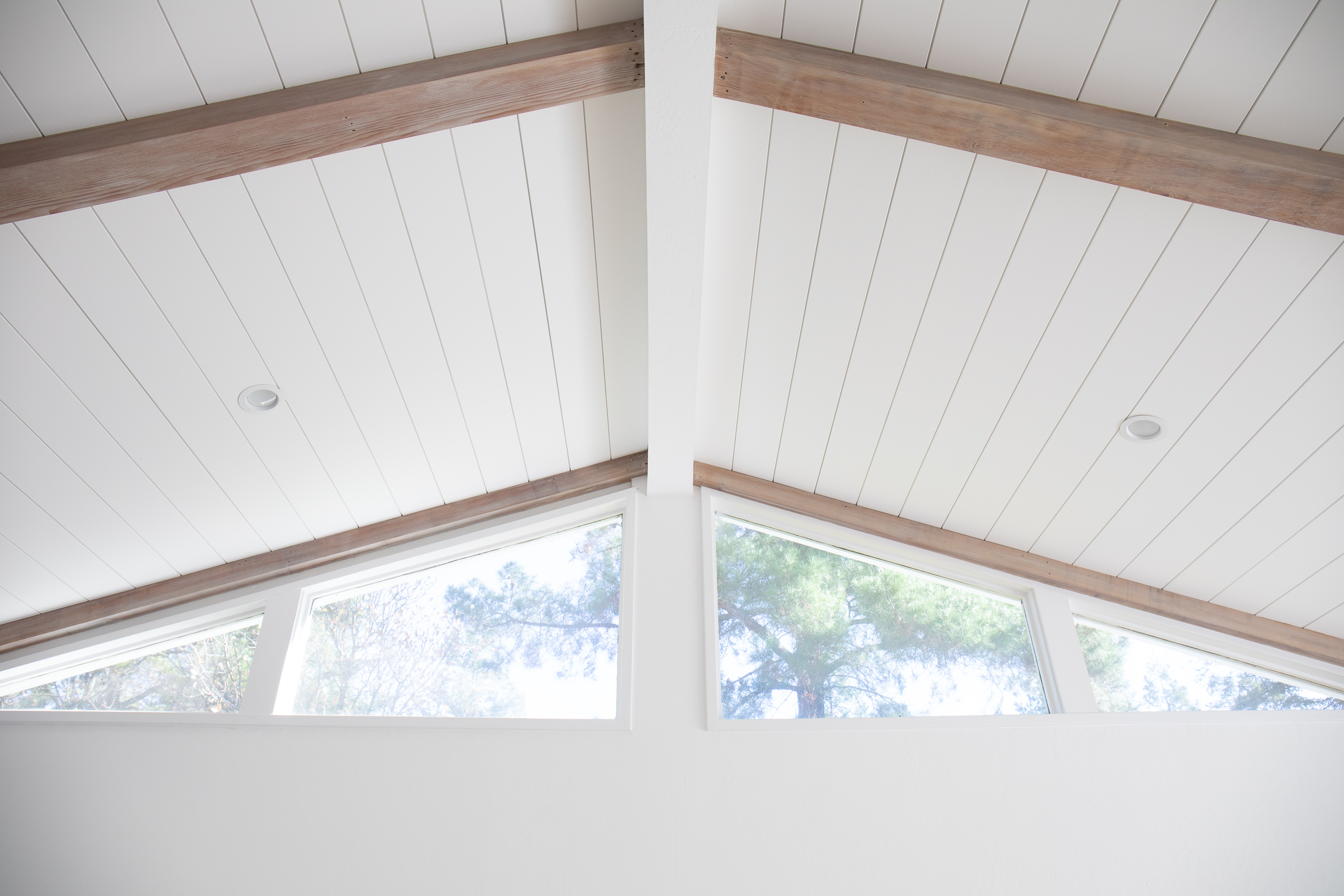This detailed image captures the interior view of a pitched, triangular-prism-style roof, characterized by its arched design. The structure prominently features white boards running across the inside, contrasted by the support of exposed, raw brown wooden beams. At the apex of the roof, a central white beam provides key structural support. The roof houses two skylights that allow ample daylight to flood the space, illuminating the otherwise monochromatic setting. Additionally, four arched windows, two larger and two smaller triangular ones, punctuate the walls, offering picturesque views of the green trees outside. This natural scene indicates that the photo was taken during a bright, sunny day. Furthermore, two light fixtures are centrally positioned but are not illuminated, further emphasizing reliance on natural light. The scene likely depicts a part of a housing or a DIY project, given the raw and unfinished aesthetic of the support beams. Overall, the image's primary colors are a stark white, earthy brown, and splashes of green from the trees outside, creating a serene and airy indoor atmosphere.